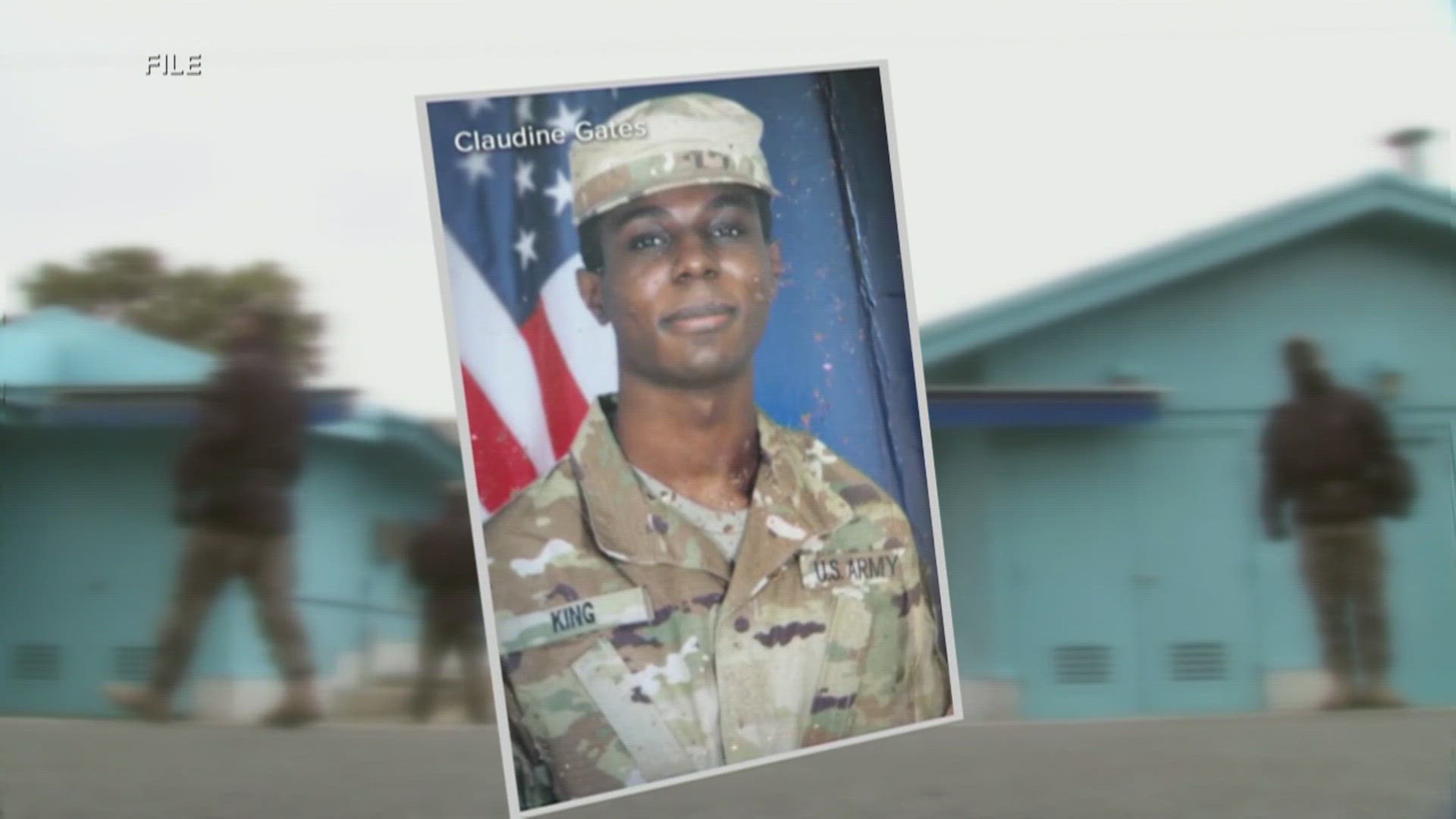In this horizontally aligned rectangular picture, the background is a blurry scene of a cloudy gray sky with two light blue buildings, each having a triangular roof. The building on the left has a tree peeking out from behind it, while the building on the right is adjacent to a fence and appears to have doors visible at the bottom. There are figures in military gear walking around; two are seen on the left and one on the right, all wearing dark-colored uniforms.

In the center of the image, a clear photo of a U.S. Army soldier is prominently displayed. This African-American soldier is smiling at the camera, wearing a green camouflage uniform with his name "King" on the right chest and "U.S. Army" on the left. He has an Army hat with a camouflaged headband. The soldier is pictured in front of an older-looking blue wall on the right and an American flag on the left. The top left corner of the photo contains the words "Claudine Gates" written in white.